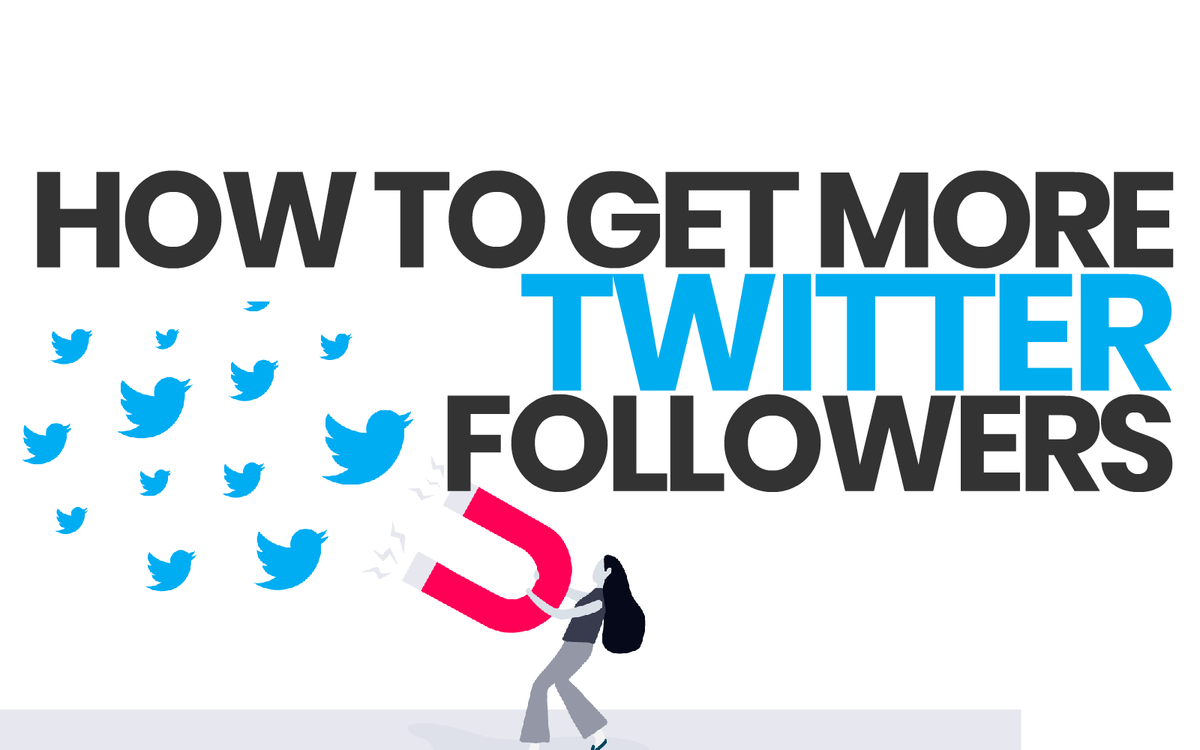Ad Illustration Description:

Centered prominently in the image is an advertisement that promotes a service designed to help individuals gain more Twitter followers. The caption "How to get more Twitter followers" takes up a significant portion of the image with the words "How to get more" and "followers" rendered in large, bold, black text. The word "Twitter" stands out, written in the signature blue color and stylized with the Twitter logo font.

Towards the bottom left of the image, an animated flock of Twitter bird logos, numbering around ten and varying in size from large to small, is depicted. These bird icons symbolize a growing number of Twitter followers, reinforcing the message of the advertisement.

In the bottom center of the image, a detailed cartoon graphic features a woman with long, flowing black hair dressed in a dark black or gray shirt paired with light gray pants. She is depicted leaning back, gazing to the left, while holding a sizable red magnet pointed upwards towards the flock of Twitter bird logos, signifying her efforts to attract more followers.

The woman stands on a simple gray bar representing the ground beneath her feet. Although her shoes display hints of color, either blue or green, it's challenging to distinguish precisely due to the limited pixel detail at the bottom of the screen. 

Overall, this advertisement serves as a visual guide or promotional piece for a social media service, potentially positioned on a website or linked to an article focused on expanding one's Twitter follower count.